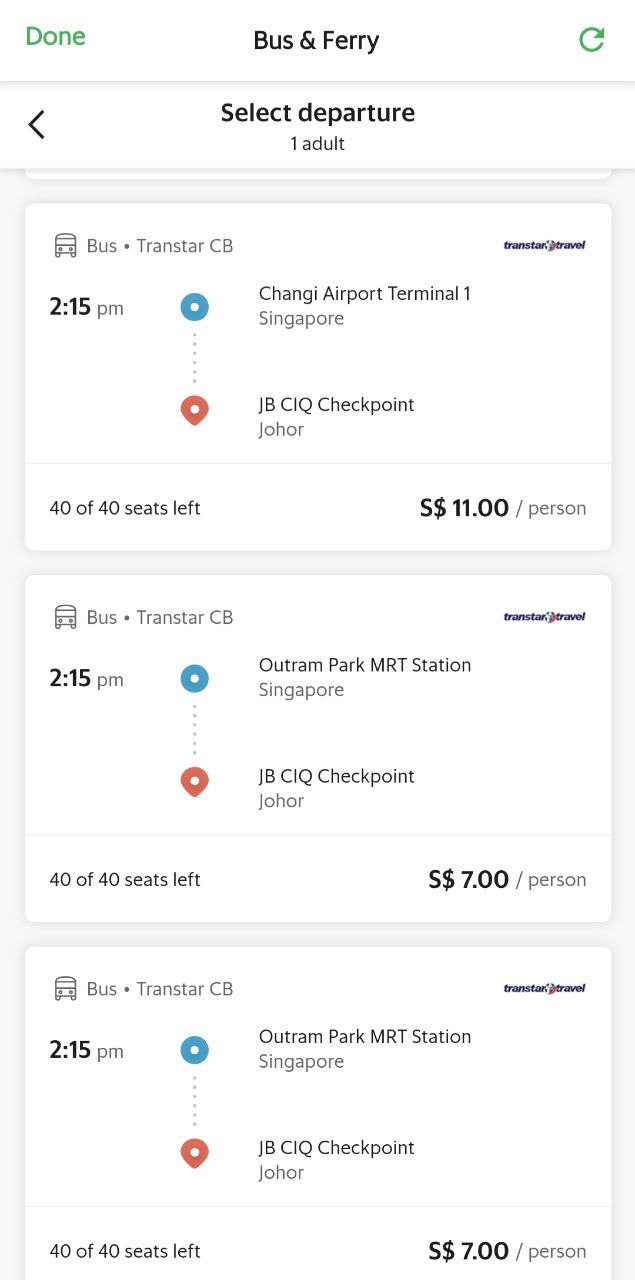This image depicts a detailed bus and ferry schedule, prominently displayed on the website. At the top of the webpage, the title "Bus and Ferry" is written in bold black text.

To the right side, there is a functional bar with a "Done" button in green and a green circle with an arrow on the right. Below that, the text reads "Select Departure" and "One Adult." The schedule starts with:

1. **Bus Transfer:**
   - **Departure Time:** 2:15 PM
   - **Pickup Point:** Changi Airport Terminal, Singapore
   - **Route:** 
     - JB Sentral Checkpoint, Johor (Symbolized with an orange circle)
   - **Availability:** 40 of 40 seats left
   - **Fare:** $11 per person
   
In the next section of the schedule, the details are as follows:

2. **Bus Transfer:**
   - **Departure Time:** 2:15 PM
   - **Pickup Point:** Outram Park MRT Station, Singapore
   - **Route:** 
     - JB CIQ Checkpoint, Johor (Highlighted with a blue circle symbol initially followed, an orange pin indicating Johor)
   - **Availability:** 40 of 40 seats left
   - **Fare:** $7 per person
   
Lastly, another similar entry:

3. **Bus Transfer:**
   - **Departure Time:** 2:15 PM
   - **Pickup Point:** Outram Park MRT Station, Singapore
   - **Route:** 
     - JB CIQ Checkpoint, Johor (Marked with an orange-yellow pin)
   - **Availability:** 40 of 40 seats left
   - **Fare:** $7 per person